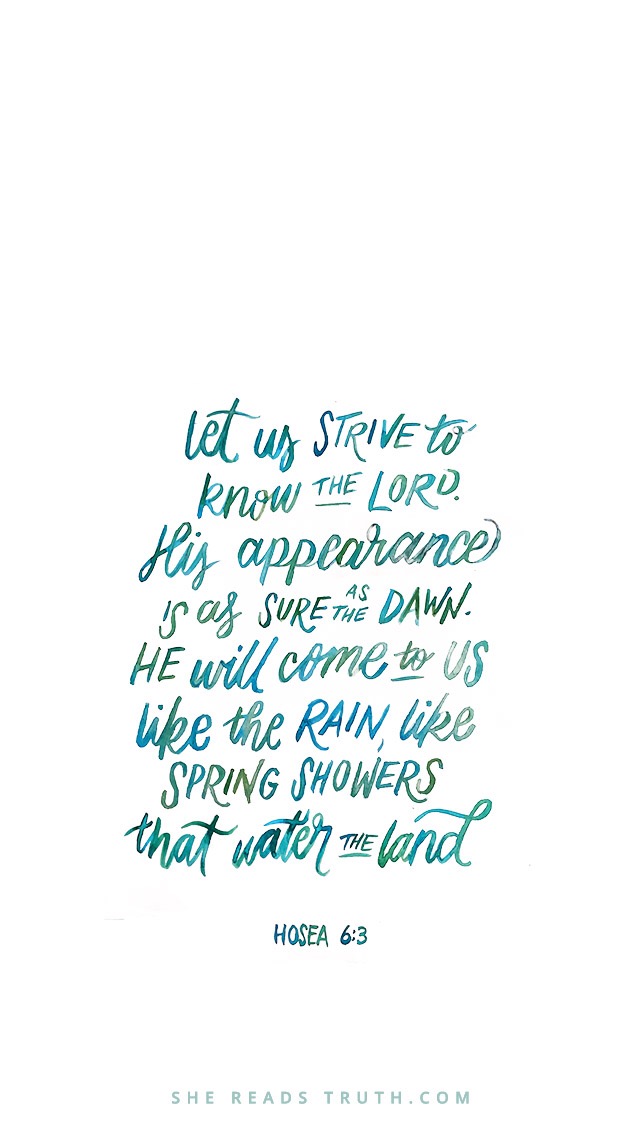The image is an inspirational graphic designed for social media, featuring a quote from the Bible on a white background. The text, presented in a handcrafted-style script that transitions between shades of green, blue, and turquoise, reads: "Let us strive to know the Lord. His appearance is as sure as the dawn. He will come to us like the rain, like spring showers that water the land." This scripture, attributed to Hosea 6:3, is displayed in a mix of cursive and curvy plain lettering, with selective capitalization for emphasis. Below the quote, in a light gray blocky font, the text "SheReadsTruth.com" is displayed, segmented as "She Reads Truth.com." The overall effect is that of a beautifully crafted religious message suitable for sharing on platforms like Facebook or Instagram.